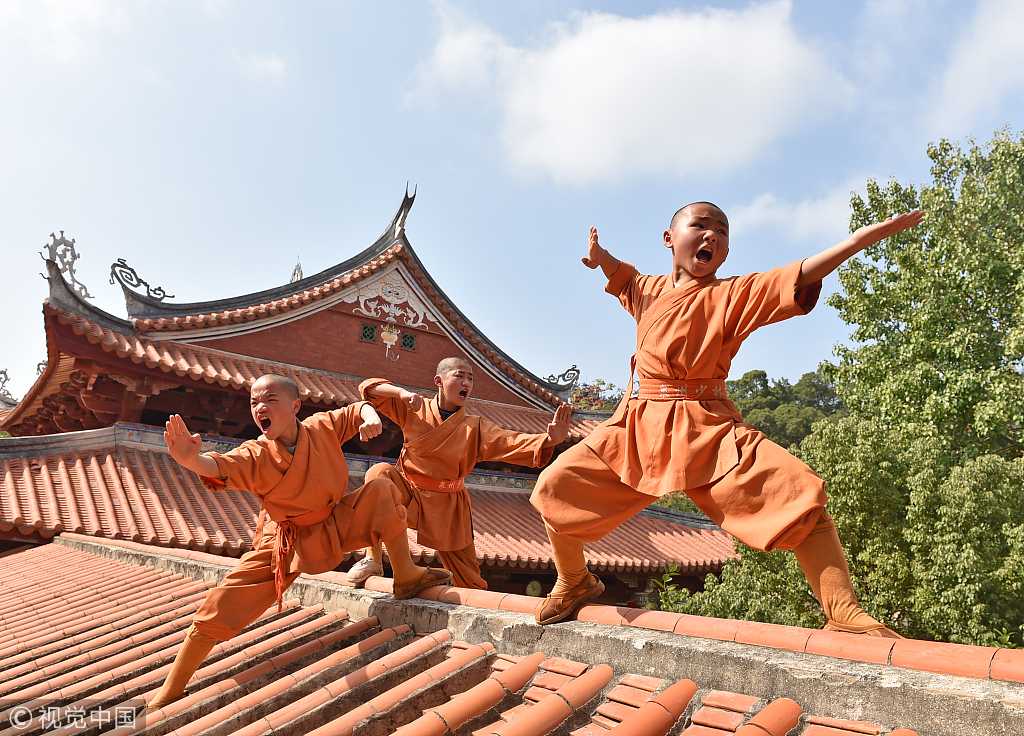The image depicts an outdoor daylight scene of three young boys posing on the rooftop of a long red building. Dressed identically in vibrant orange kung fu outfits, complete with sashes and low-lying leather boots, the children adopt exaggerated martial arts stances, hands raised and feet spread, as though in mid-action. Each boy has a shaven head and seems to be shouting, enhancing the dynamic energy of their poses. The rooftop is adorned with red brick, tile roofing, and in the background rises a slightly taller, more compact red building with decorated higher roof peaks featuring stylized dragons on each of the four corners. Green treetops peek from behind the taller structure, extending into a vast sky dotted with a few fluffy white clouds. In the bottom left corner of the photograph, there is a gray box with white text, indicating a copyright symbol followed by four non-English characters, possibly Chinese or Japanese.